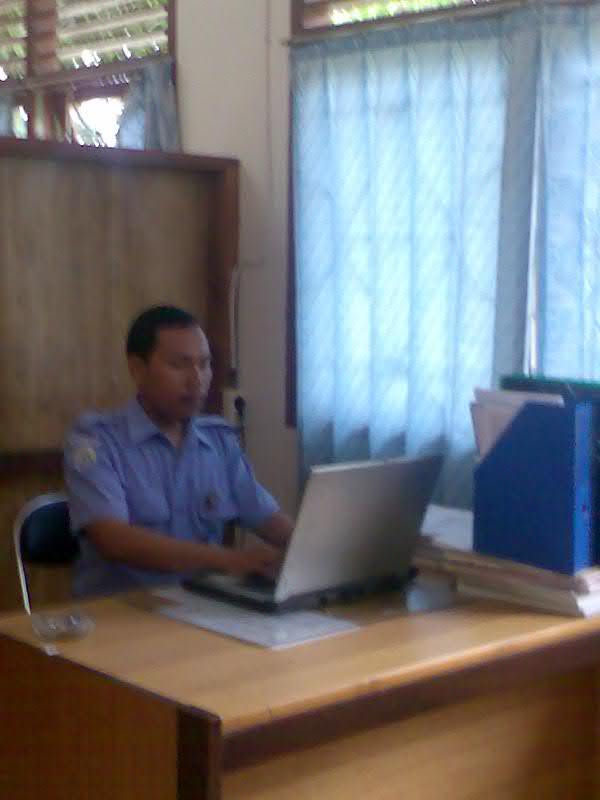The photograph captures a young man with dark hair and a dark complexion, intently working at a brown wooden desk that is situated by a window adorned with cheap, perfunctory blue curtains. The man appears to be wearing a blue uniform, possibly indicative of a police officer or some other government official. His shirt features lapels on the shoulders and likely a badge attached to the breast pocket, with a patch or pin on his right arm. He is focused on a laptop with a silver top and a darker bottom, surrounded by stacks of papers and a bright blue folder. Behind him is a wooden partition separating his cubicle-like space, and above it, there seems to be additional windows. The setting suggests he is at work, diligently performing his duties.